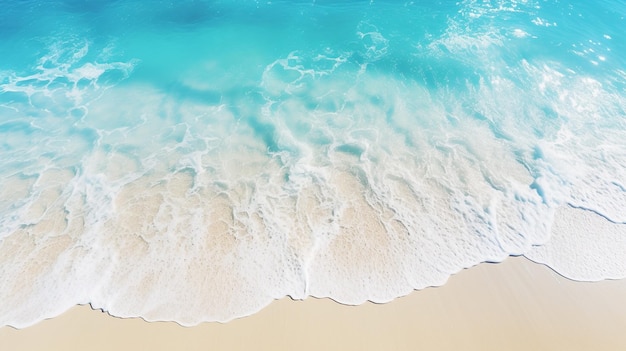This aerial photograph captures the mesmerizing interaction between the ocean waves and a pristine, beige-colored sandy beach. The image, likely taken from a drone or airplane, offers a high vantage point, showcasing the expansive and remarkably smooth shoreline. The turquoise blue, crystal-clear water transitions gracefully into a thin, white, gauzy foam as the waves approach and spread out onto the flat, untouched sand. The sunlight reflecting off the deep blue-green water enhances the vibrant colors and highlights the gentle flow of the tendrils of water reaching the beach. The photograph is bordered by a clean, white edge, framing the scene beautifully and making it a perfect candidate for wall display. The overall composition emphasizes the captivating natural gradient from the turquoise ocean to the white foamy waves, and finally to the smooth, beige sands, creating a serene and striking visual spectacle.